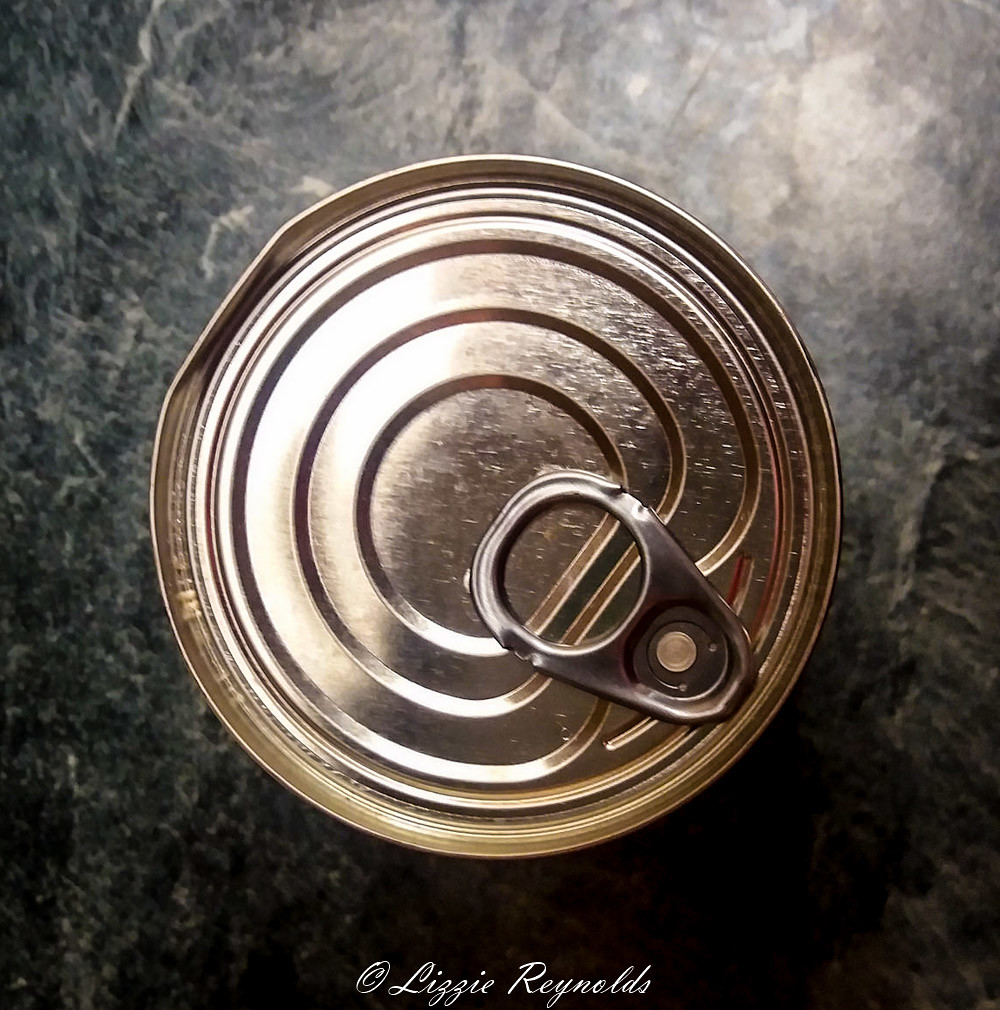In this image, a gold tin can is prominently displayed on a table with a black surface featuring white and gray textures. The tin can is positioned with its bottom resting on the table, and the photograph is taken from a top-down perspective. Notably, the top left of the can is slightly bent. The can lid is adorned with gold rings, and there is a silver handle located on the bottom right. This handle, used for opening the can, has a hole at its end. At the bottom of the image, white text can be seen, reading "See copyright: Lazy Reynolds" from left to right.